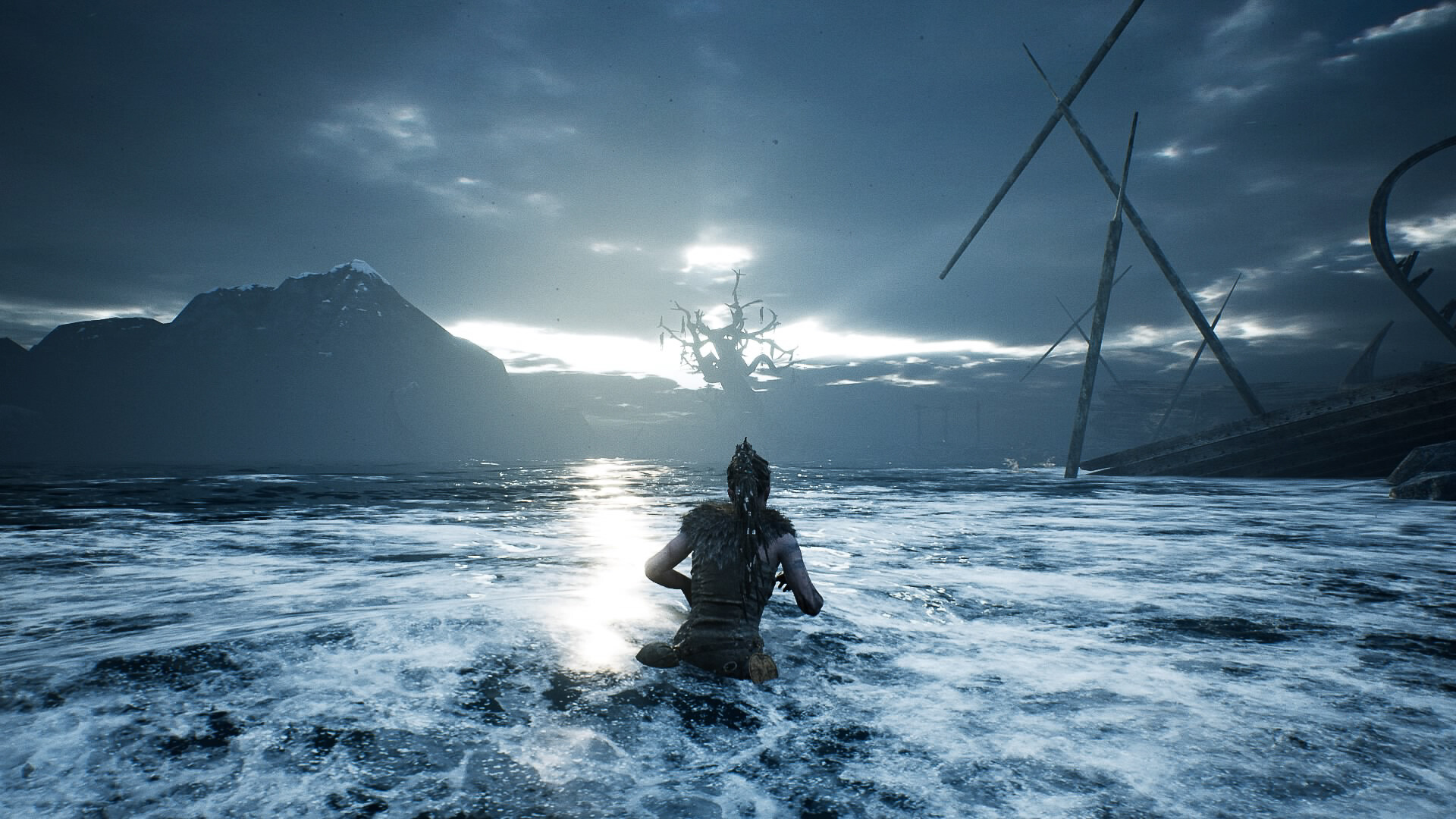In this surreal and dramatic scene, a lone figure wades through frothy, turbulent ocean waters, their back turned toward the viewer. They wear a fur-type outfit with short sleeves and have long hair, leaving their gender ambiguous. The churning, white-capped sea lacks distinct waves yet seems violently agitated. To the right, the remnants of a shipwreck are visible, its masts jutting out at precarious angles, partially submerged. The distant horizon is a spectacle of dark storm clouds parted by a burst of sunlight, casting an ethereal glow on the water's surface. Adding to the surrealism, a gnarled, bare-limbed tree inexplicably rises from the clouds, and a looming, snow-capped mountain appears to emerge from the sea itself. The juxtaposition of these elements - the ocean, shipwreck, radiant sun, tree, and mountain - suggests this image is an AI-generated or heavily manipulated creation rather than a still from a movie, capturing a fantastical vision that defies natural laws.